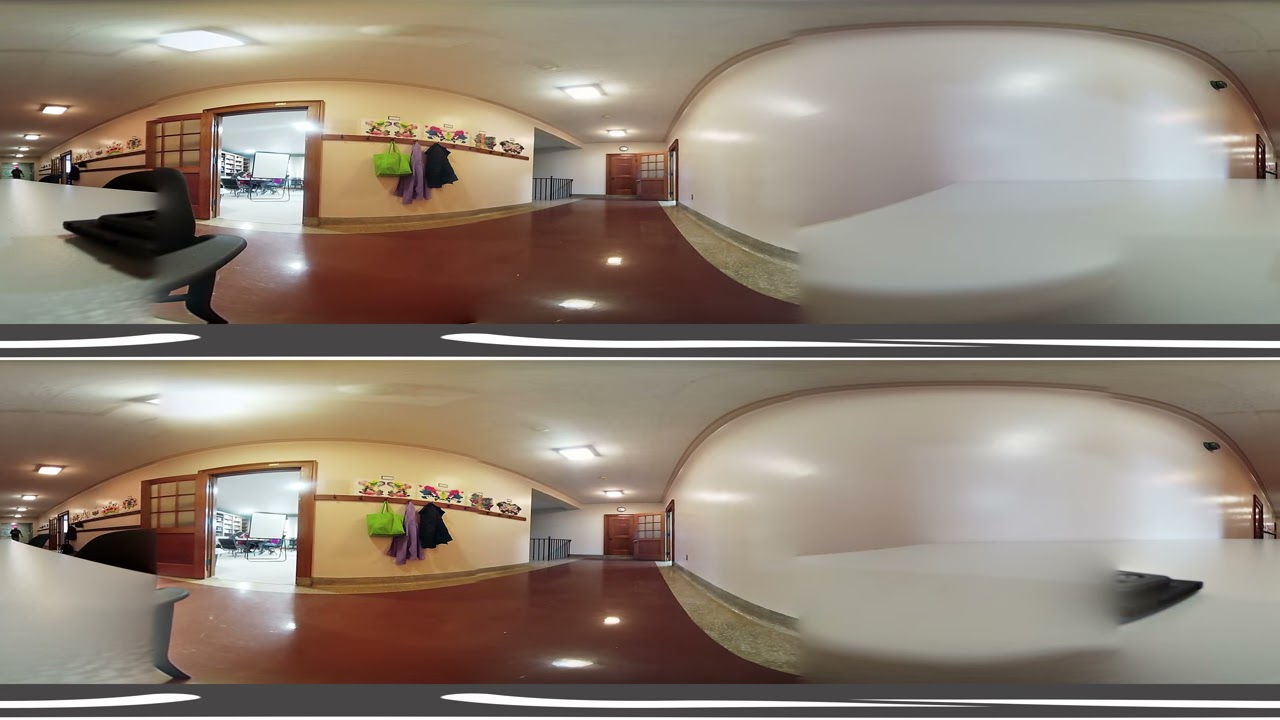This composite image features two nearly identical panoramic photographs, one positioned above the other. Both images capture a detailed view of a school hallway characterized by light tan walls and a shiny dark brown floor that reflects fluorescent lighting. On the left side of the images, an open door reveals a brightly lit classroom equipped with desks, tables, and a centrally located whiteboard. Inside the hallway, hooks on the wall hold a neon green handbag or backpack, a purple coat, and a black coat. A notable difference between the two photographs is the presence of a black office chair in the upper image, positioned just in front of the classroom door, while in the lower image, the chair seems obscured by distortion. Additionally, there is a wooden-framed beige wall with a checkered window or door next to it and a shelf bearing various items protruding from the left side. The right side of both images features a frosty white oval shape that appears blurred out, suggesting missing or indistinct details in this section of the hallway.